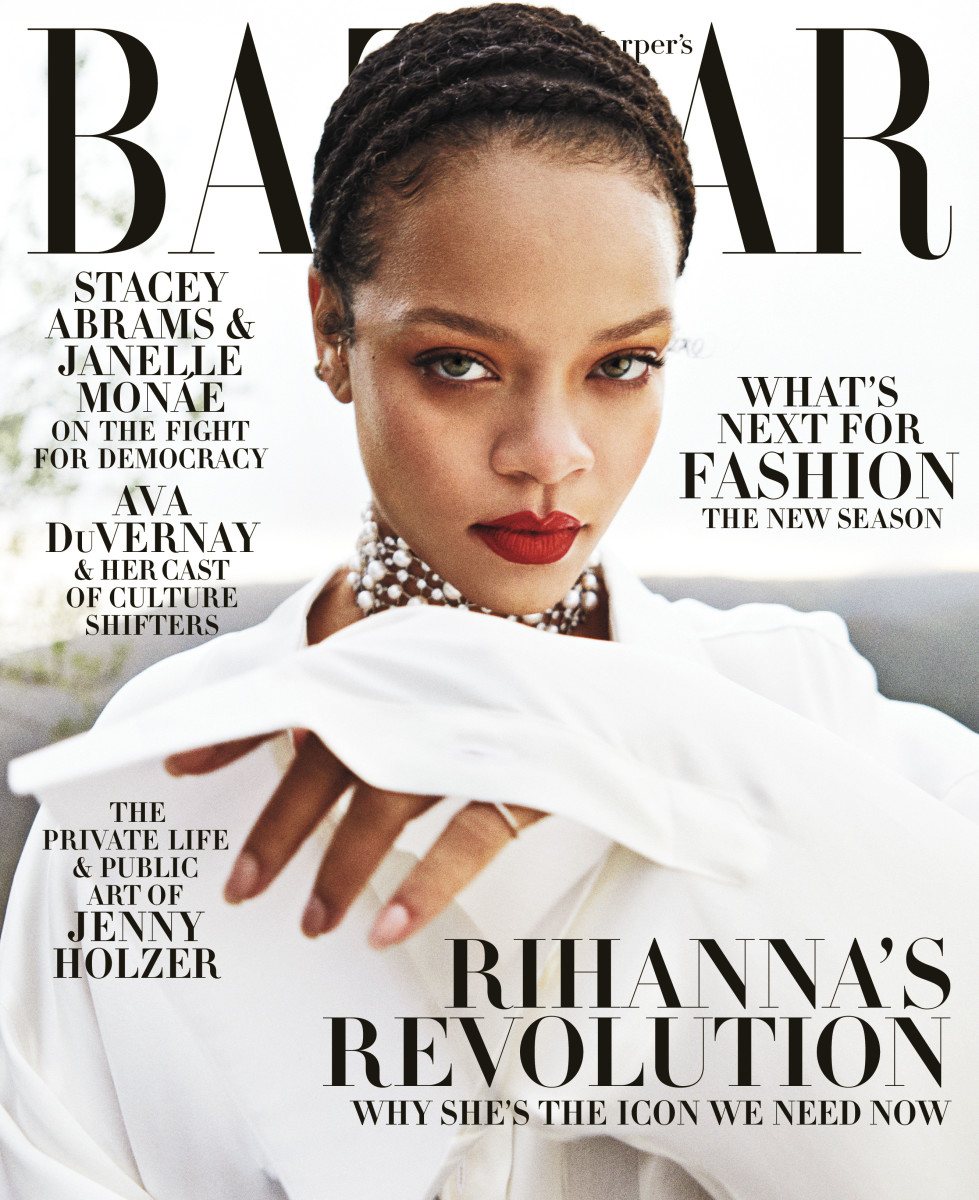On the cover of a magazine titled "BAAR," we see a striking portrait of a woman with dark hair styled in intricate braids that loop around the top of her head. She has red lips and her eyes, which are directed towards the camera, convey a sense of calm intensity. Her full face is visible, featuring a composed expression without a smile. She is adorned with a white necklace and a white long-sleeve shirt, evoking a pristine and elegant appearance. Her left hand is raised towards the front of the image, showcasing a ring on her pinky finger. 

The bottom of the cover features bold text proclaiming "Rihanna's Revolution: Why She is the Icon We Need Now." On the right are the words "What's Next for Fashion: The New Season," hinting at future trends in the industry. The left side includes articles titled "Stacey Abrams and Janelle Monáe on the Fight for Democracy" and "Ava DuVernay and her Cast of Culture Shifters." Additionally, the bottom left corner teases an insightful piece on "The Private Life and Public Art of Jenny Holzer."